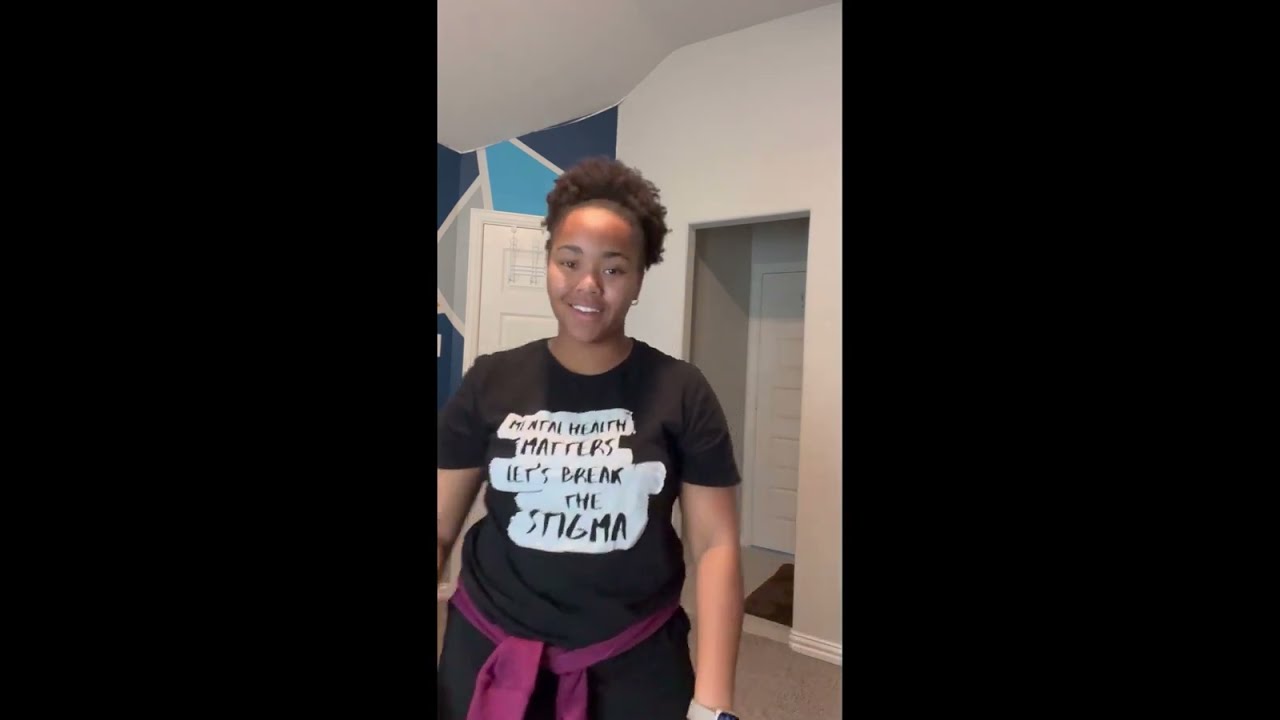A smiling Black woman stands in the center of the image, which is divided into three sections, with the woman occupying the middle third. She wears a black t-shirt with the slogan "Mental Health Matters: Let's Break the Stigma" written in white, handwritten-style text on a black and white cloud-like background. Her attire is completed with black pants and a burgundy sash tied around her waist. She has natural curly black hair, pulled back into a loose ponytail. The background reveals an off-white wall and ceiling, with a blue geometric design consisting of light blue, dark blue, and gray shapes on the wall partially visible through an open door on the right. The open doorway exposes a brownish wall outside, a shadow falling across the scene, and a light-colored carpet in the adjacent room with a darker patch on it. The left and right sides of the picture are framed by black borders, adding contrast to the image's composition.